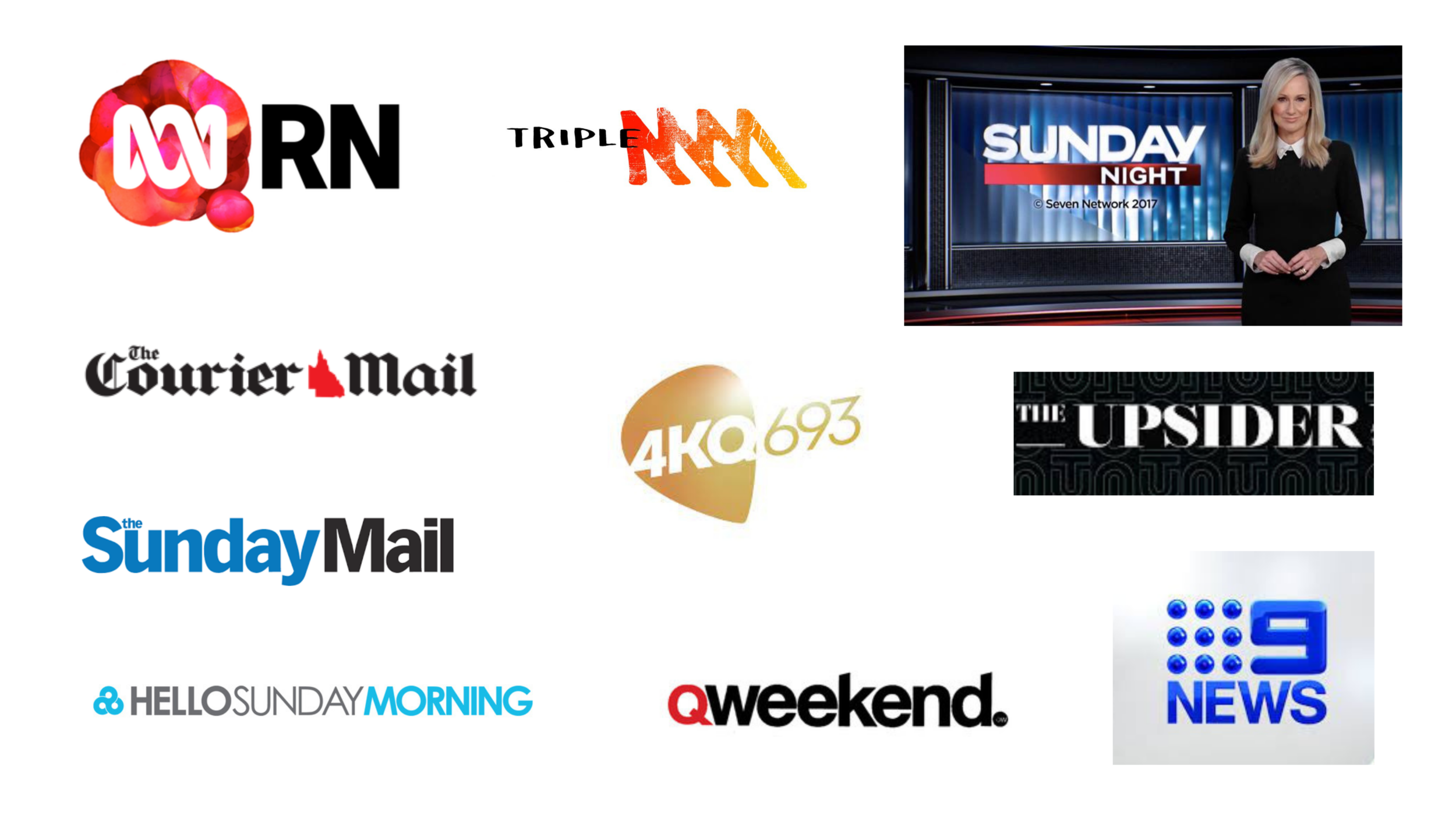This image displays a collage of various media logos arranged on a white background. In the top left corner, there is a logo for RN. Centrally featured is an art logo for Triple M, while on the far right, a thumbnail for Sunday Night Seven Network shows an anchor standing beside a TV. Additionally, the collage includes logos for The Courier-Mail, 4KQ, 4KQ693, The Upsider, The Sunday Mail, Hello Sunday Morning, QWeekend, and 9 News. The first and second rows each contain three icons, while four icons are positioned at the bottom.